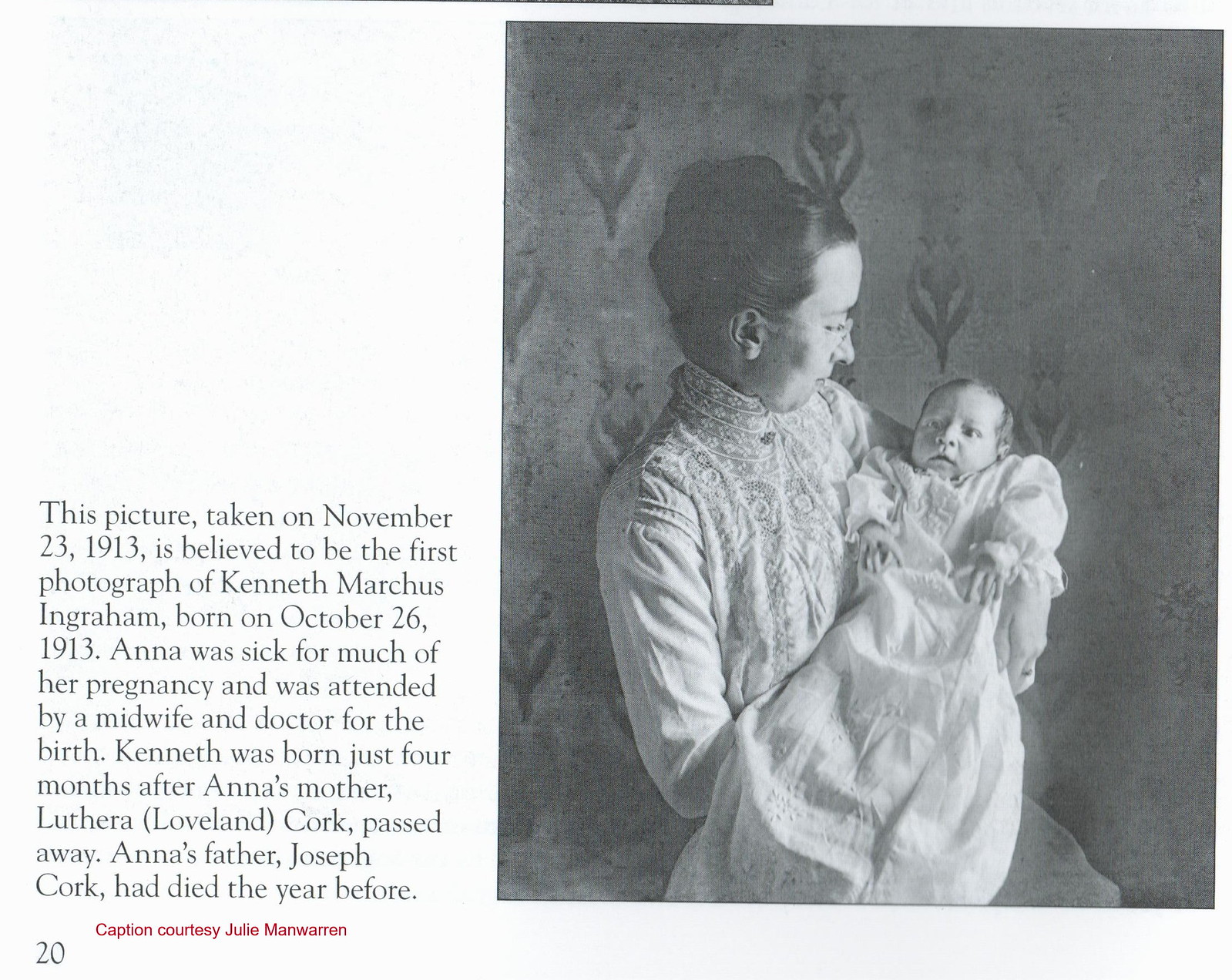The photograph is a black-and-white image on the right side of a wide rectangular format. It depicts a woman with slicked-back hair styled in an updo, wearing a long-sleeve lacy outfit and holding an infant on her lap. The baby, appearing frightened, is dressed in a long white gown with its hands forward and face towards the camera. The background features a floral patterned wallpaper. The detailed caption to the left, in black text, states: "This picture, taken on November 23rd, 1913, is believed to be the first photograph of Kenneth Marches Ingraham, born on October 26th, 1913. Anna was sick for much of her pregnancy and was attended by a midwife and doctor for the birth. Kenneth was born just four months after Anna's mother, Luthera Loveland Cork, passed away. Anna's father, Joseph Cork, had died the year before." Additionally, in red text in the bottom corner, it reads: "Caption courtesy of Julie Mann-Warren," with a notation of "page 20".